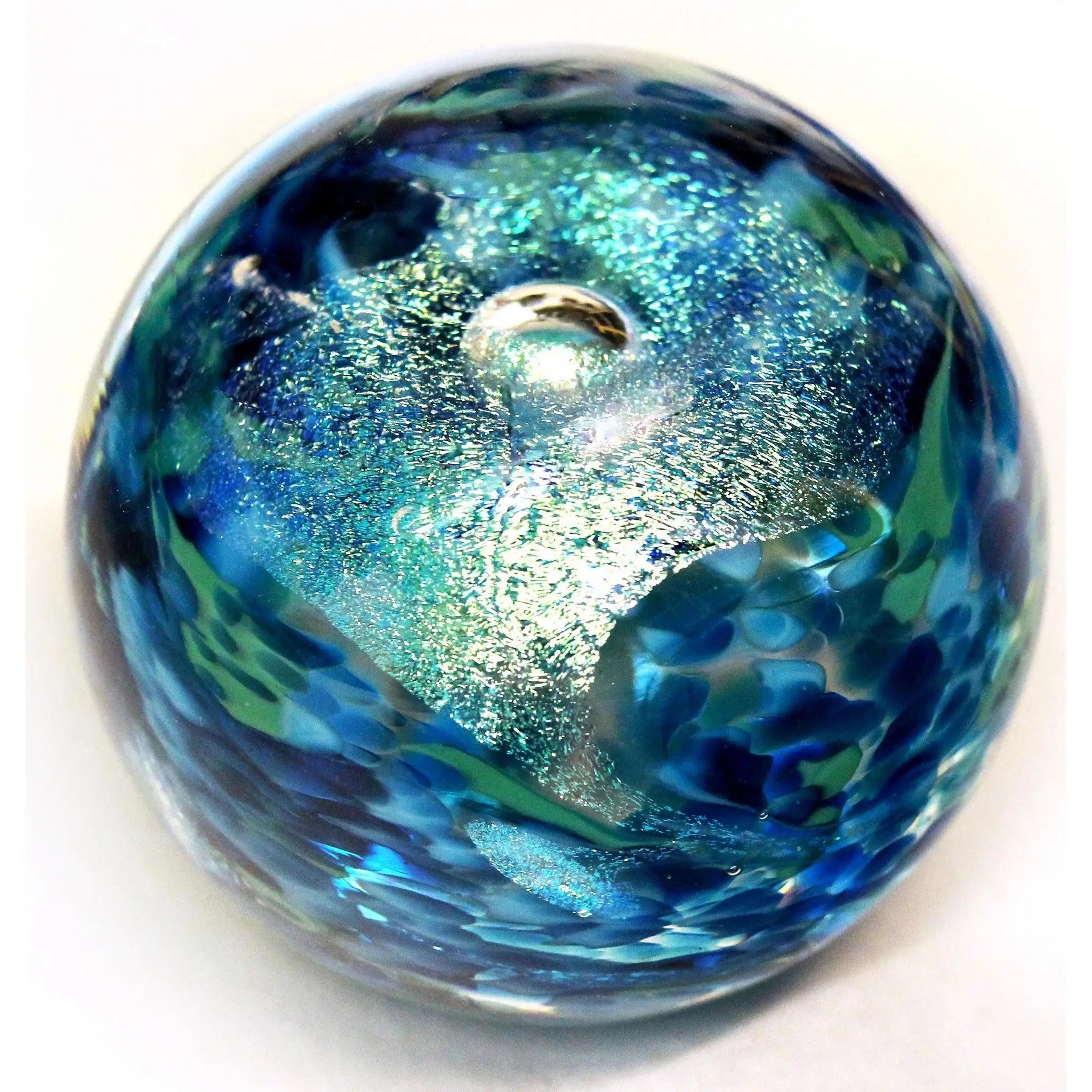The image features a glass globe-like paperweight set against a light cream or white background. The globe exhibits a stunning mix of colors and textures, including dark blue, light blue, turquoise, and green, all arranged in round splotches and swirls, making the surface mottled and dynamic. At the top of the globe, there is a clear, crystal-like section that appears to have an iridescent layer and resembles a bright sunburst, complete with reflective qualities showing a shimmer of colors like silvery and gold. Another focal point is a clear bubble within this section that captures and reflects light from the surrounding environment. The entire object exudes a shiny and glossy finish, making it remarkably eye-catching and intricate.